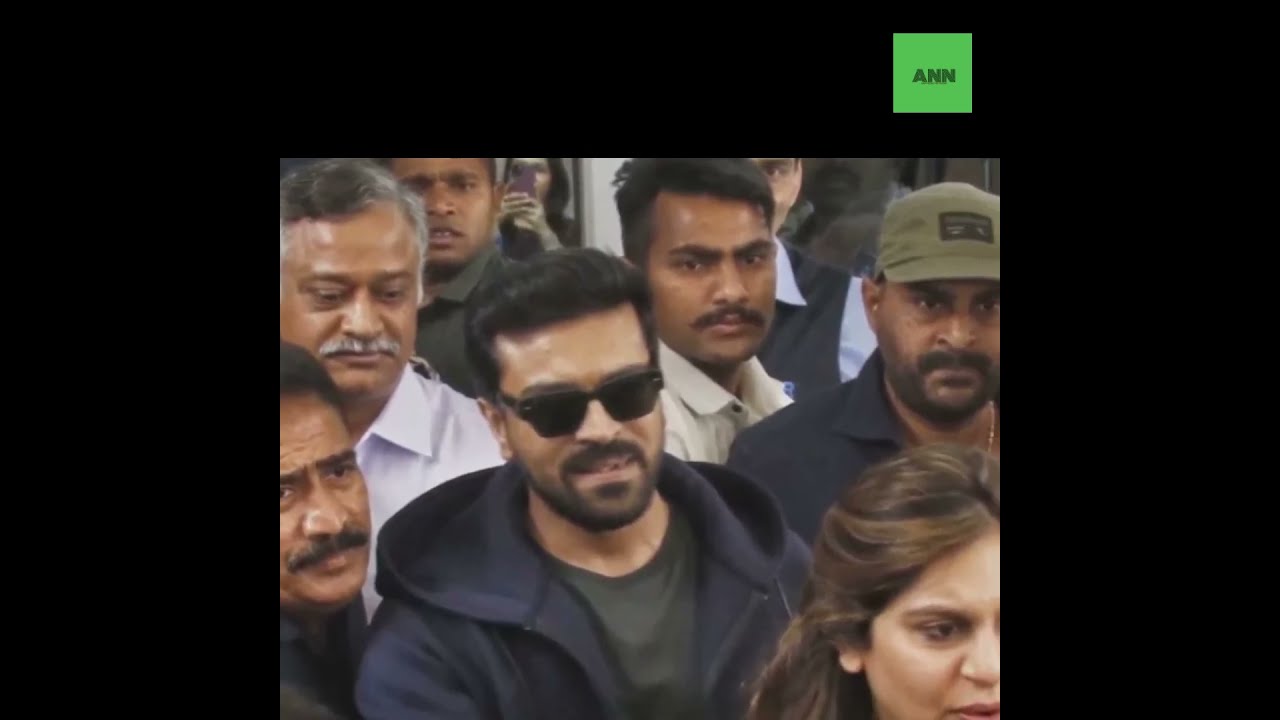A detailed image depicts a group of about seven South Asian individuals, gathered closely together and seemingly forming a small crowd focused around a central figure. The person in the center, possibly in his 30s, stands out with his dark sunglasses, neatly trimmed black facial hair, and a combination of a dark blue zip-up hoodie over a gray t-shirt. His attire and demeanor draw immediate attention, hinting at his possible celebrity status, potentially being escorted by his companions. The group includes a range of individuals: directly in front of him is a concerned-looking brunette woman with her hair half back, while to his left stands a middle-aged man with short black hair and a black mustache, donned in a black shirt. An older man with salt-and-pepper hair and a gray mustache wearing a white shirt stands slightly behind them. To his right are two men; one wearing a green baseball cap and a black goatee, dressed in a black shirt, and another man with dark sunglasses and a black beard, sporting a gray shirt. The people appear to be facing the camera, their expressions varying from neutral to slightly worried, and exhibit a sense of casual style. The photograph is bordered in black on the sides and top, with a green rectangle containing the letters "A-N-N" in black text in the upper corner.